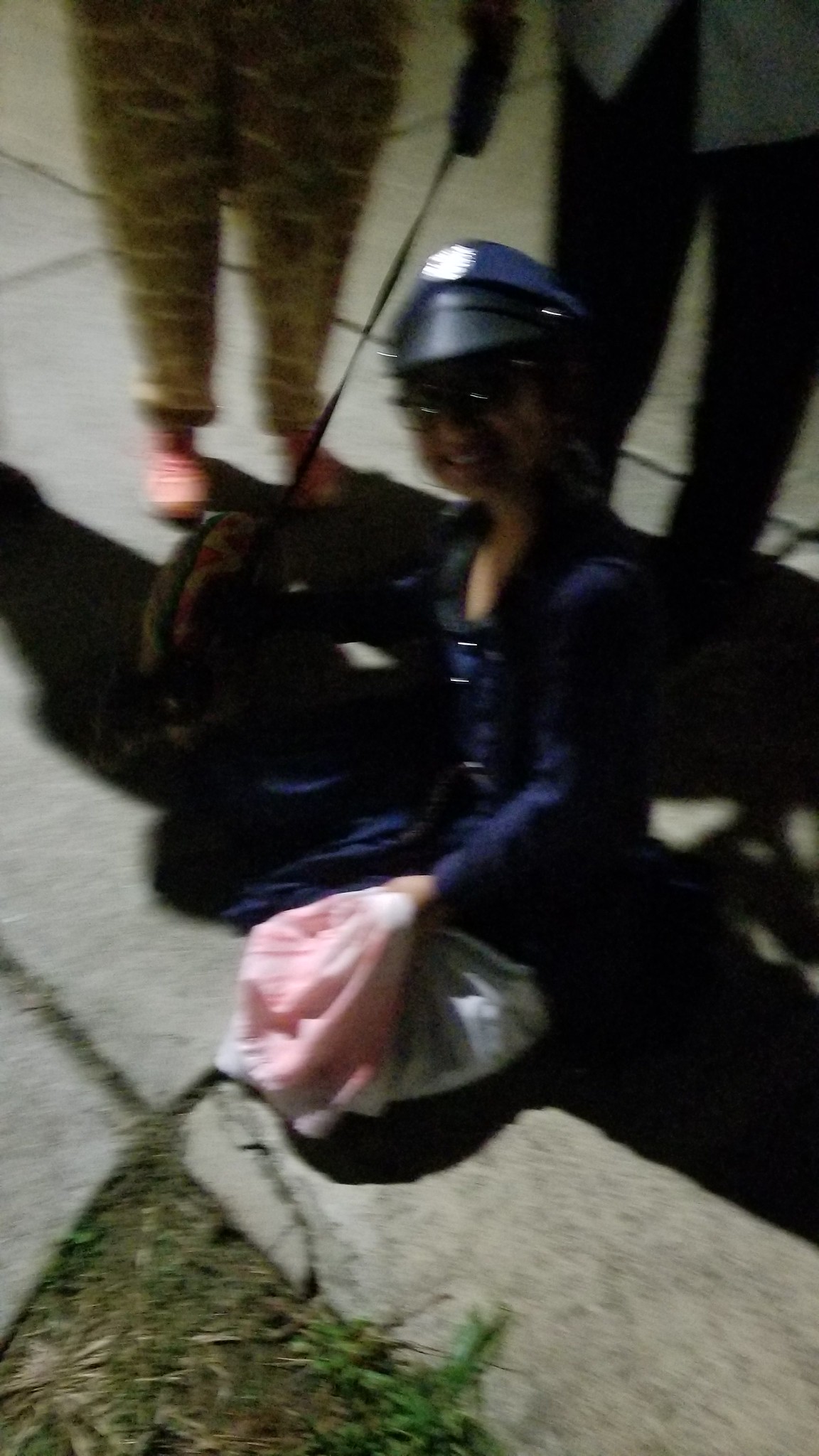The image depicts a nighttime scene illuminated by a distant light source, possibly a streetlamp, casting shadows on a sidewalk divided by patches of dirt and sparse grass. At the center, a woman is seated on the concrete, dressed in a navy blue uniform with a hat that features a shiny badge on its leather brim, suggesting she might be in some sort of official or costume attire. She holds a bag that is white with pink accents, indicative of either a tote or a purse. To her right, there appears to be luggage on the ground. Behind her stands another individual in dark pants and a white shirt or jacket, holding an object that might be a leash, though no dog is visible due to the image's poor lighting. Additionally, another person in the background is partially visible, wearing camouflage pants and distinctive pink running shoes, adding to the scene's eclectic mix of attire.